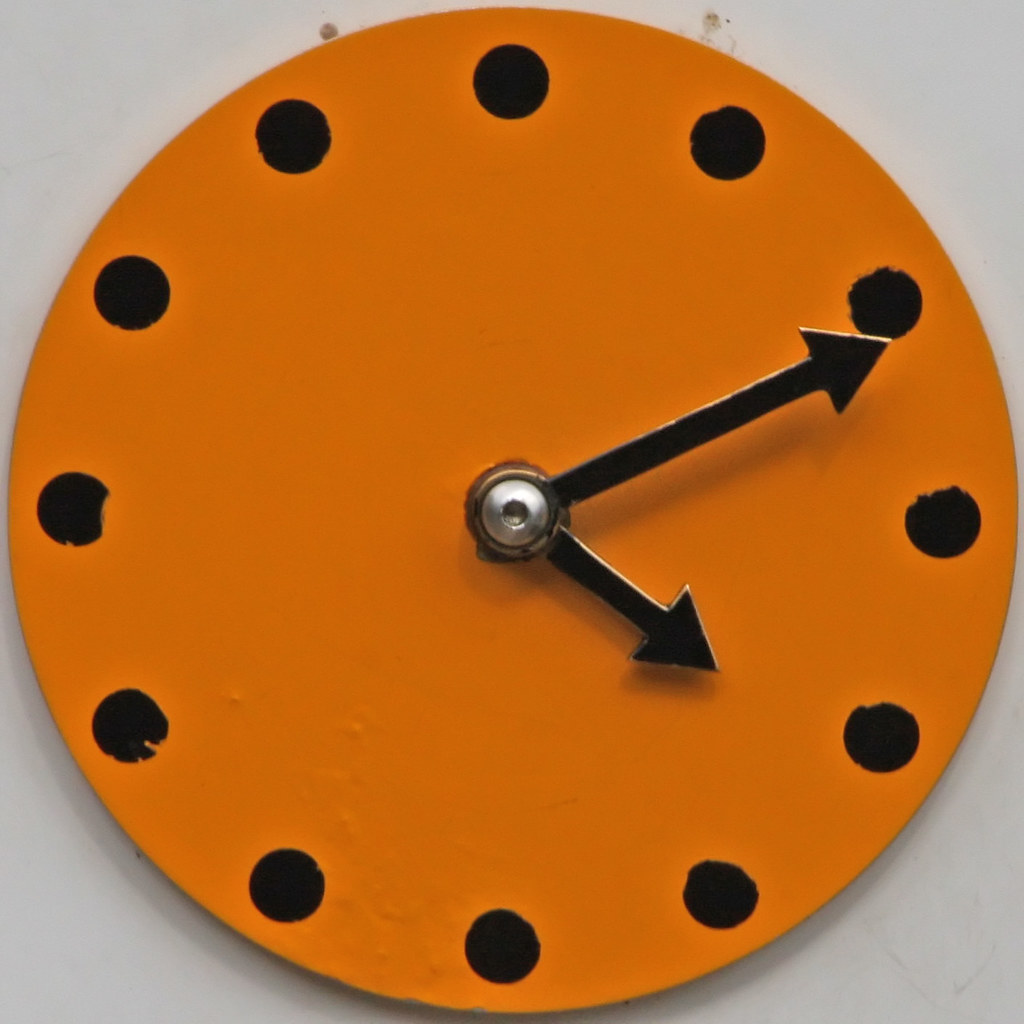This close-up image depicts a simple, circular clock with a distinct orange face mounted against a white background, likely a white wall. The clock is meticulously painted, although evident brush marks hint at some areas where the paint is slightly worn off. Instead of traditional numbers, black filled-in circles mark the hours, some of which appear imperfect and faded. The clock hands, also black and shaped like arrows, are securely fastened to a central, dome-like silver screw with an indent in the middle. The longer minute hand points to where the 2 o'clock position would be, while the shorter hour hand points slightly past 4, indicating the time as 4:11.